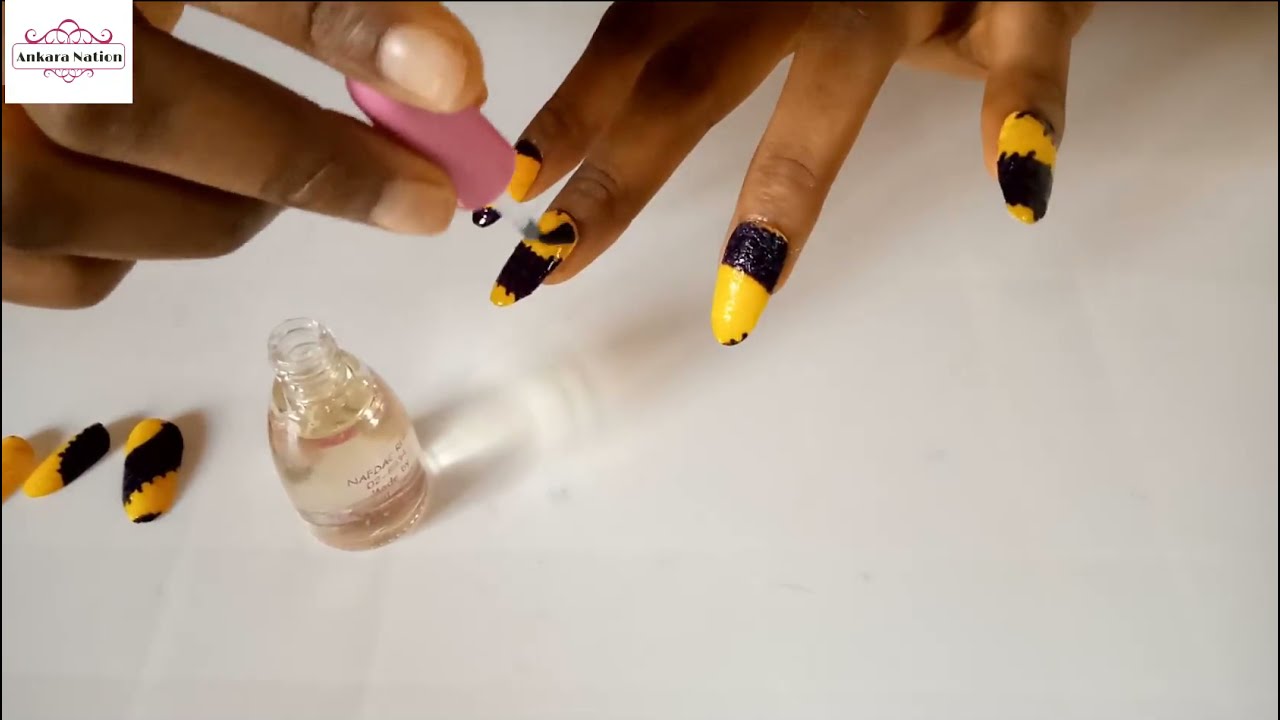In the image, we observe a wide rectangular scene featuring a girl with dark brown skin meticulously painting her nails at a table. Her right hand, which holds a pink-handled nail polish brush, is applying a clear coat to her nails, one of which is already adorned with a striking yellow and black pattern. The left hand is visible holding the nail polish brush, with its fingernails still unpainted. Scattered on the off-white tabletop are additional black and yellow patterned fake nails, ready for application, along with a small bottle of clear or pearl-colored nail polish. In the upper left corner, the image bears the text "Ankara Nation" alongside a distinctive pink logo featuring curls and circles. Shadows cast lightly on the surface, adding depth to the detailed ritual of nail art being performed.